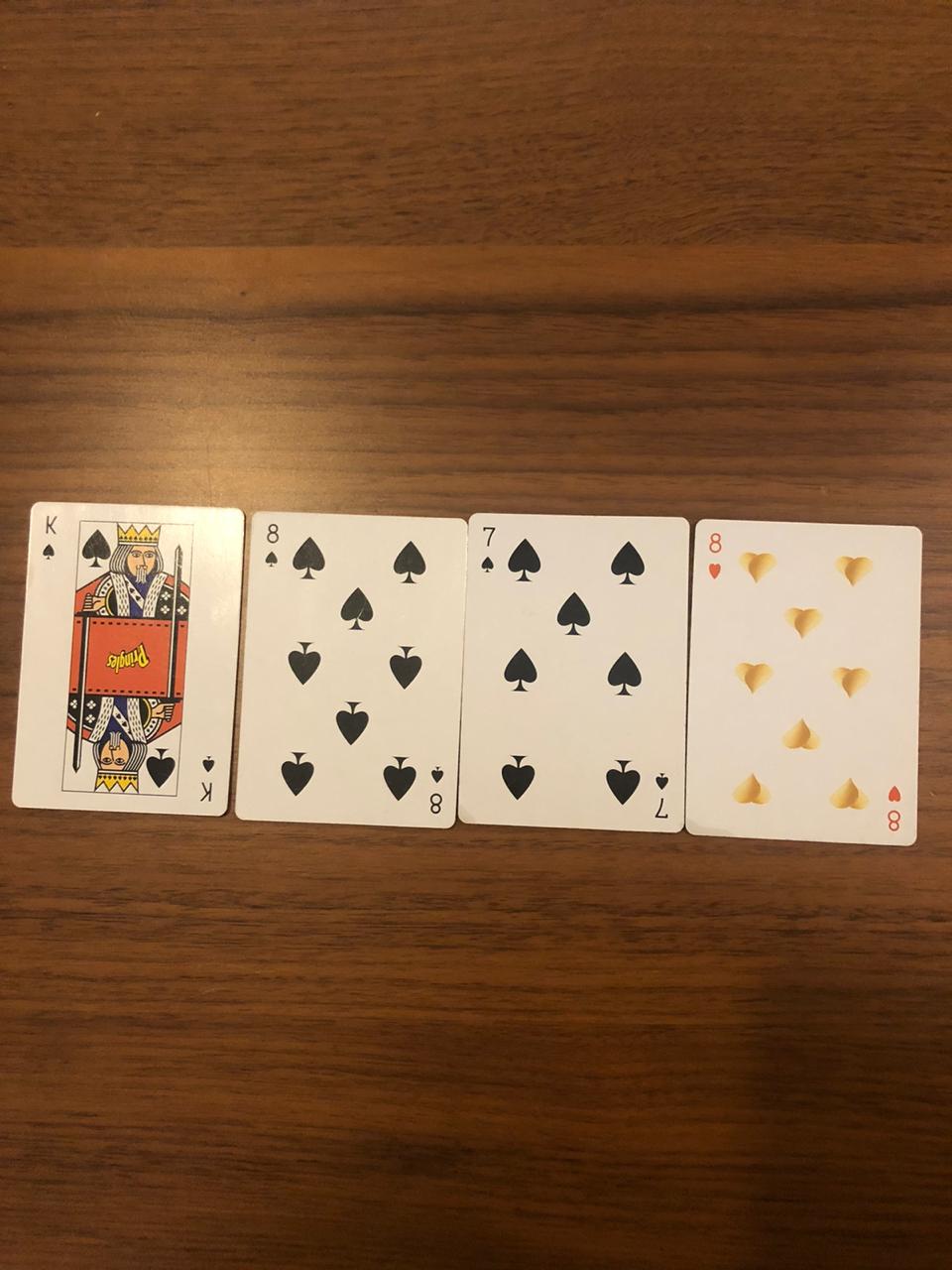This photograph showcases four vintage playing cards meticulously arranged on a grainy wooden table with an equally textured wooden backdrop. The cards on display are the King of Spades, the Eight of Spades, the Seven of Spades, and an intriguingly unique Eight of Hearts adorned with eight intricately designed fish instead of the traditional heart symbols. The King of Spades, with his timeworn appearance, features a detailed illustration of a crowned monarch. His chin-length hair and pronounced beard, coupled with elaborate silver scarves, impart a sense of antiquity. The card also depicts a scepter and a spade, with two mirrored images of the king, one in an upright position and the other inverted. The entire scene exudes a nostalgic charm, capturing the essence of bygone eras.